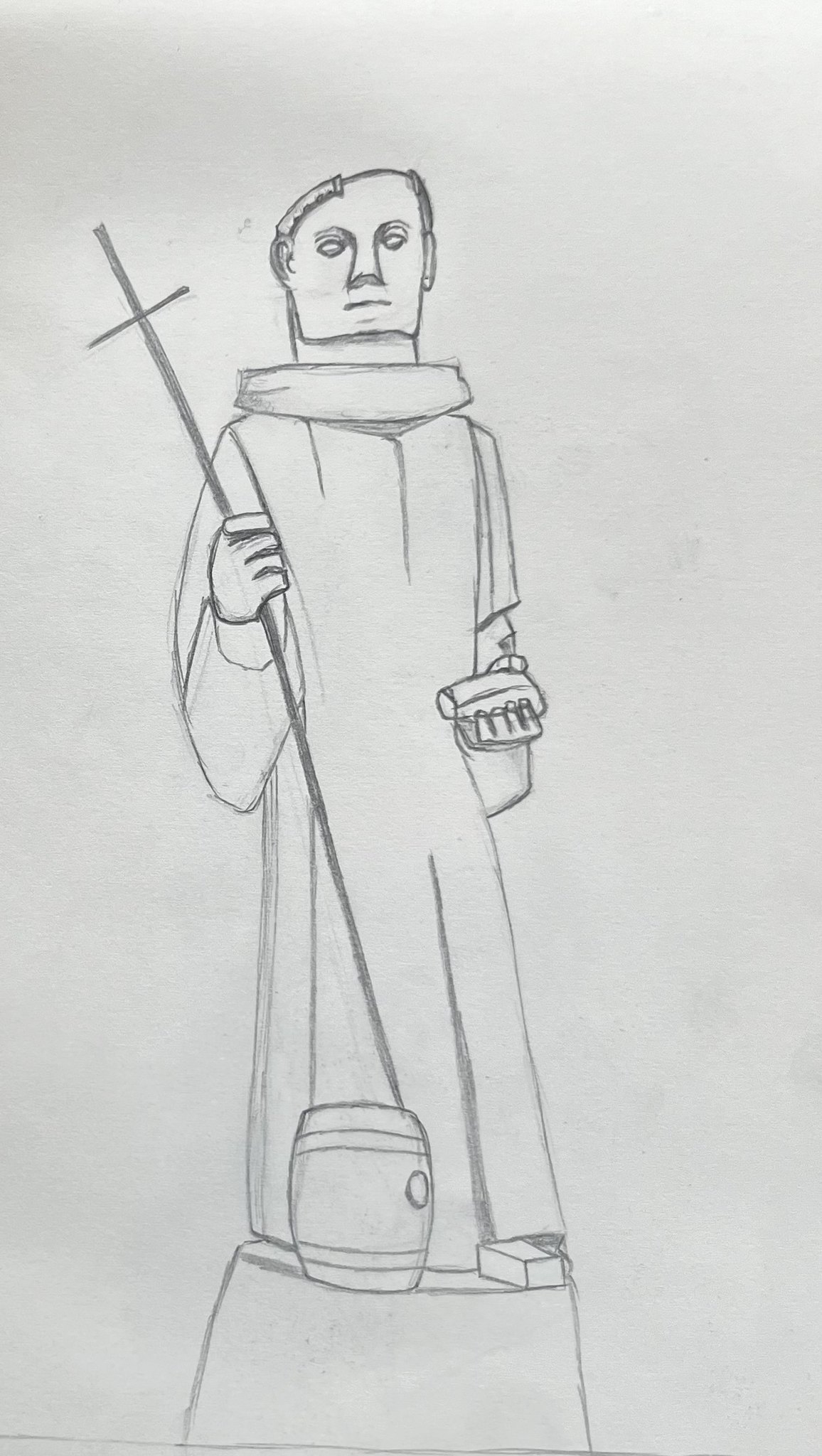This detailed vertical pencil drawing on white paper depicts a monk or religious figure standing solemnly. The figure is adorned in a long, flowing robe, indicative of monastic attire, and he holds a staff topped with a cross in one hand. The other hand grasps an indistinct object, adding an element of mystery to the scene. At his feet lies a barrel, accompanied by another rectangular object placed nearby. The monk is positioned on a platform, emphasizing his stature and significance within the composition. His facial features are minimalistic—a few strands of hair, a wide nose, and a simple line for a mouth—yet they effectively convey a contemplative expression. A collar is distinctly drawn at the top of his robe, detailing his ecclesiastical garment. The entire artwork is rendered in shades of graphite gray, contrasting starkly against the white paper, emphasizing the artist's meticulous pencil work.